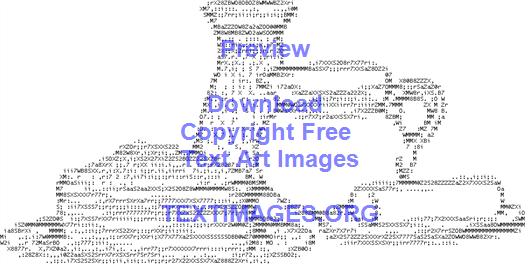The image features a white background with intricately arranged black letters forming various objects: on the left, there's a plate with a wedge of cheese, and on the right, a plate with a stick of butter. In the background, one can see a pitcher and a glass water container, both also created from numerous letters. This piece of text art is detailed, with each food item and object clearly distinguishable amidst the letter formations. Superimposed over this meticulously crafted ASCII art is a visible watermark in blue text reading, "Preview Download Copyright-Free Text Art Images - textimages.org." The overall composition is centered and displays a mix of clear and dotted letter designs to emphasize different parts of the image.